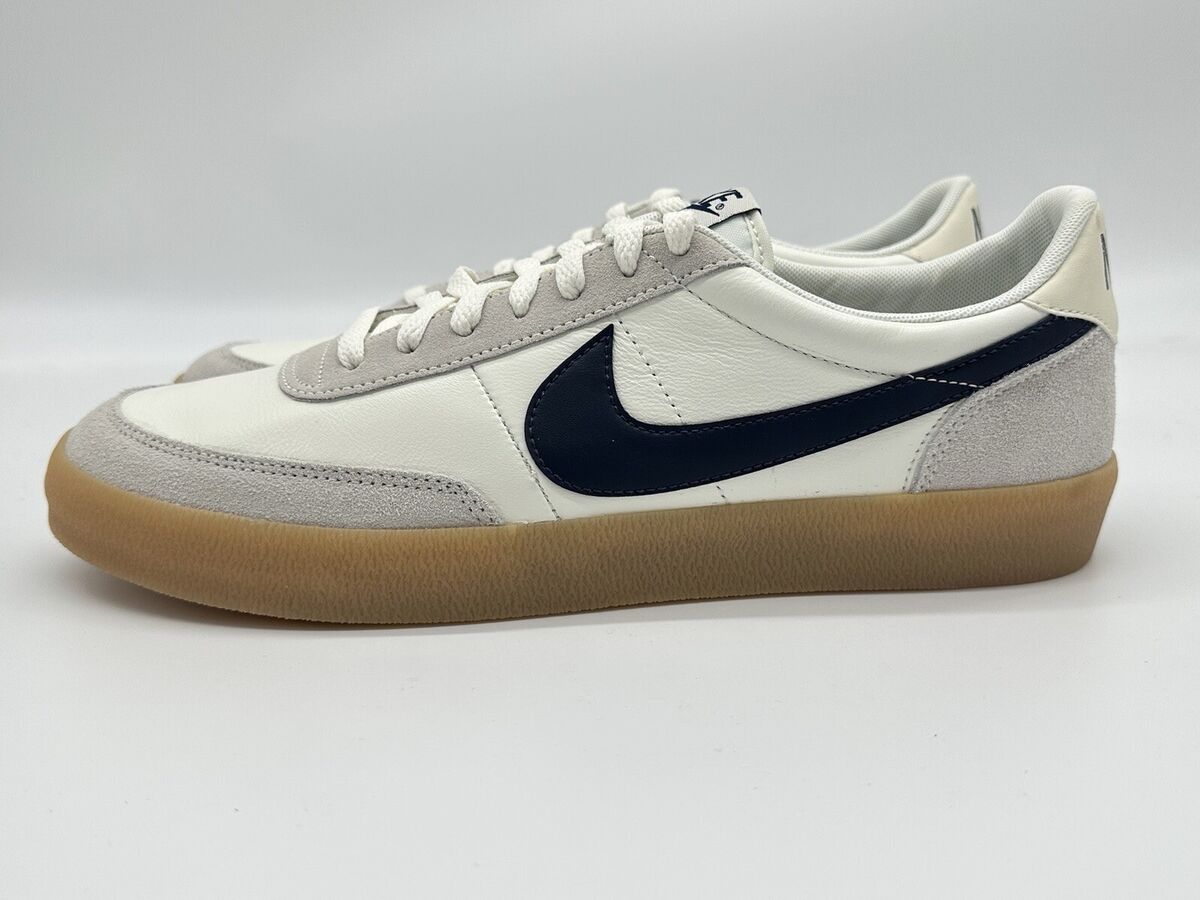This image features a pristine pair of Nike sneakers prominently displayed against a seamless white background. The sneakers, positioned to highlight the left shoe, are showcased from a side angle, accentuating the iconic black leather Nike swoosh that extends from the midsection to the heel. The upper part of the shoes is crafted from soft white leather, complemented by light gray suede trim around the toes, heel, and lace area. The laces are an off-white color, coordinating with the white leather tongue, which features a barely visible Nike tag at the top. The interior lining of the shoe is light gray, and the brown rubber sole adds a subtle contrast to the overall design. Only the edges of the right shoe are visible, hinted by the heel and toe peeking out from behind the left shoe. The sneakers appear to be unworn, maintaining a flawless appearance that suggests they are likely a men's size 10 or 11.